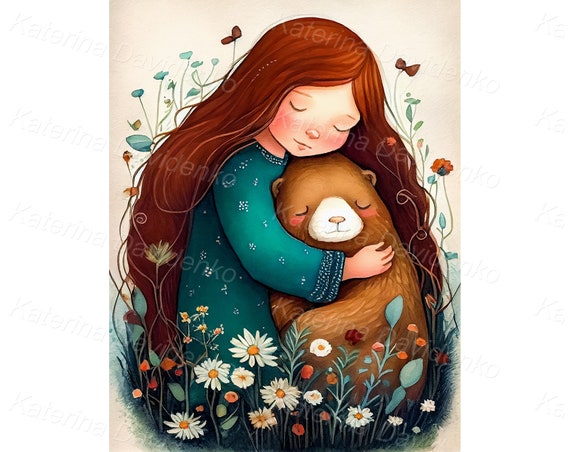In this beautifully detailed painting by the artist Katerina Devenko, a young girl with waist-length, wavy brown hair is depicted sitting in a lush field of flowers and plants. She is wearing an oversized green dress, adorned with little white dots and beads around the wrists and neck. The girl lovingly hugs a small baby bear with a distinctive white face, brown fur, a white nose outlined in yellow, and adorable red blushes under its eyes. Both the girl and the bear have their eyes closed, sharing a tender moment. Among the vibrant foliage that frames the scene, a variety of flowers—including daisies, orange, and blue blossoms—add to the enchanting atmosphere. Tall green stems and leaves frame the sides and bottom of the image, enhancing the serene, natural setting.